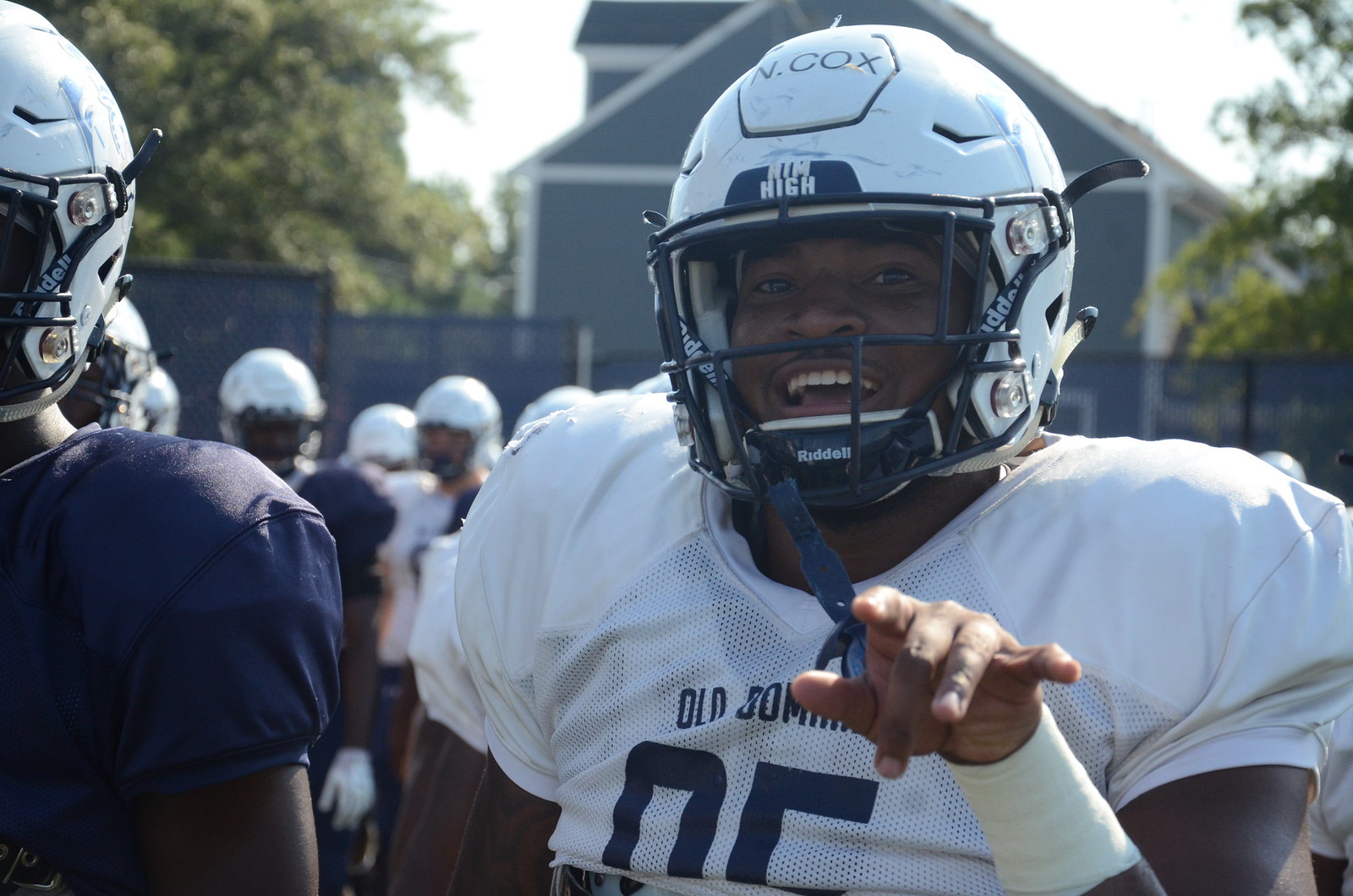In this vibrant photograph, an African-American high school football player stands out in his full gear, radiating joy as he points towards the camera with a cheerful smile. Donning a white helmet marked with "N COX" and a matching white jersey with the name "Nim High" visibly emblazoned in navy lettering, he exudes confidence and enthusiasm. His uniform is complemented by a black facemask and a white wristband on his left arm, possibly serving as a sweatband. To his right, another player in a blue jersey and white helmet makes an appearance, adding to the scene's dynamic energy. The background showcases a bustling field with players wearing both white and blue jerseys, all equipped with white helmets. A gray building enclosed by fencing hints at the outdoor setting, under a sky that appears slightly overcast. The overall atmosphere is charged with the lively spirit of high school football.